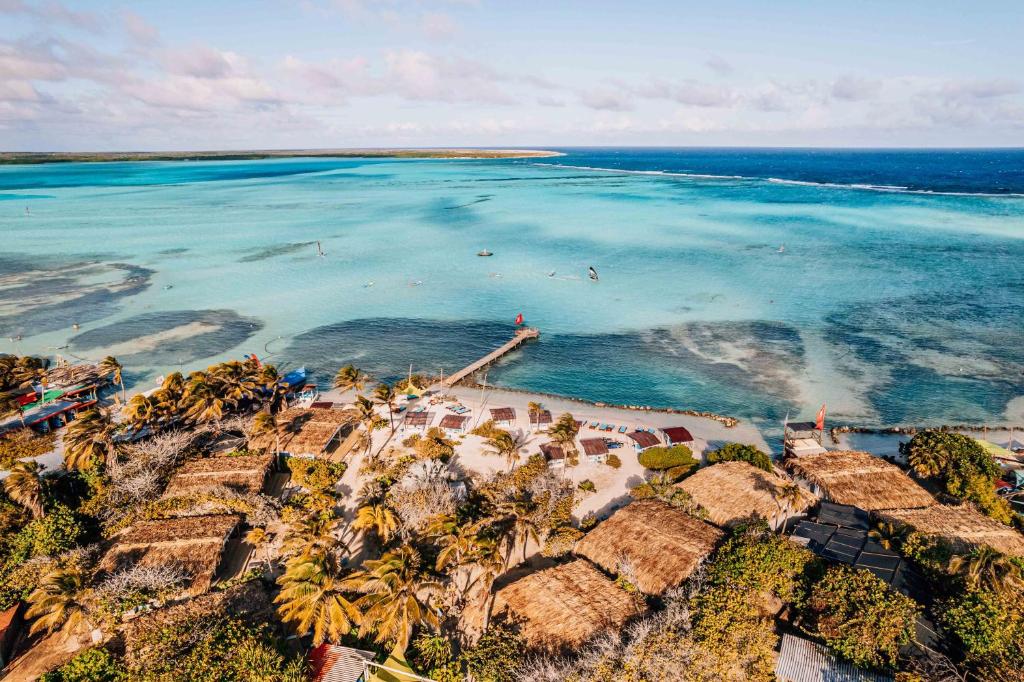The image showcases a breathtaking aerial view of what appears to be a resort on a picturesque Pacific island. Bright white sandy beaches flank the edge of a serene, crystal-clear sea that transitions from a near see-through turquoise in the shallows to a deeper, darker blue towards the horizon. Sandbars and ocean vegetation are visible beneath the shallow waters. A long dock extends into the ocean, with a person seemingly present on it, adding to the tranquil atmosphere. 

The beach is populated with several thatched-roof huts providing shade, surrounded by rows of gently swaying palm trees and lush tropical vegetation, indicating it's a windy day. Larger huts, likely accommodations for guests, nestle amidst the greenery. Bright pops of color include what may be a painted boat and colorful structures or flags, possibly marking storefronts or small buildings near the shoreline. The landscape is uninhabited, with no people visible except potentially on the dock, enhancing the peaceful, untouched feel. 

The photograph, most likely taken from a drone or aircraft, captures a scene of pure tropical beauty, complete with clear skies, vibrant waters, and rich greenery, epitomizing an idyllic island retreat.